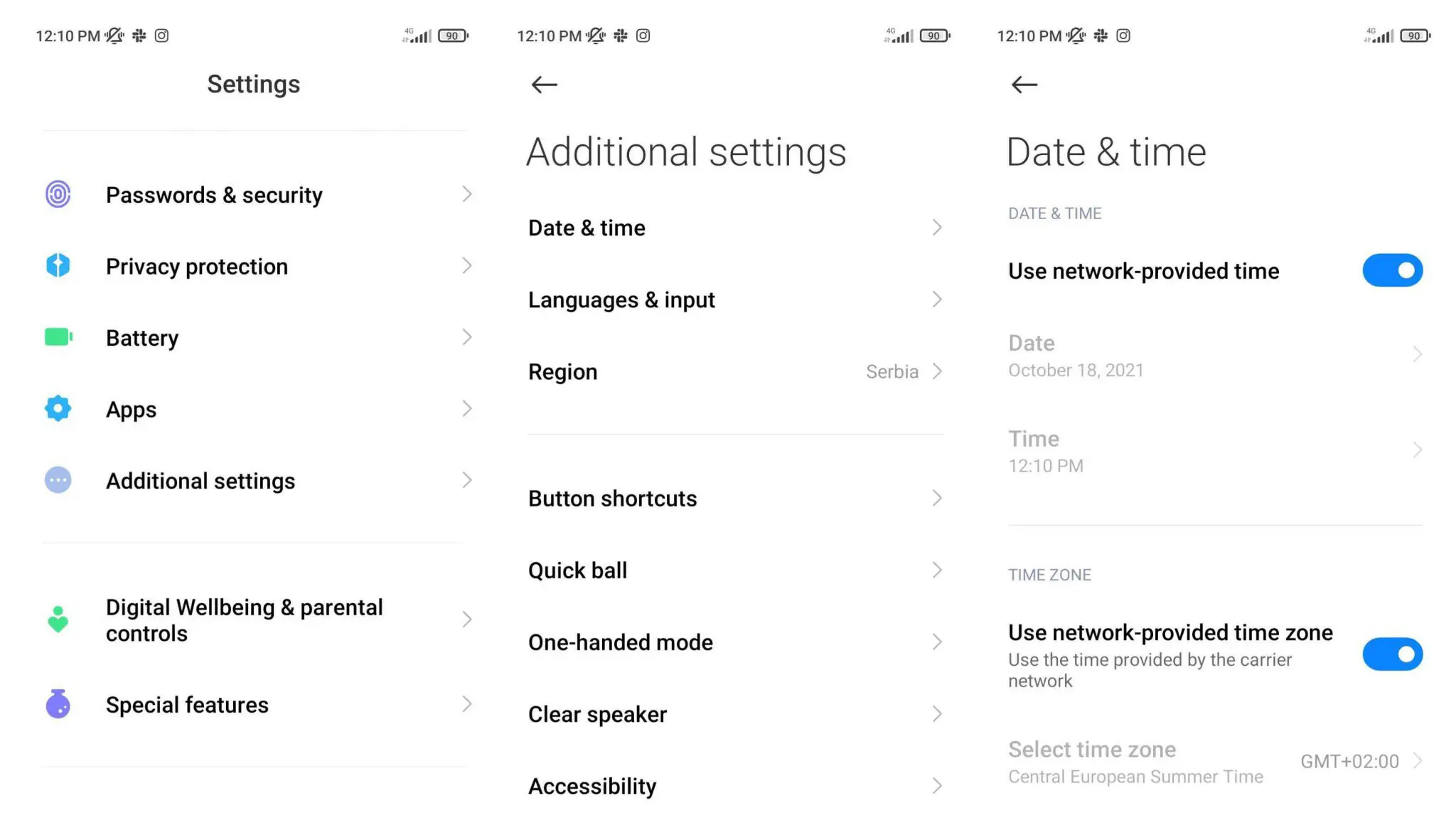This image displays a sequence of three screenshots taken on a mobile device, all captured at precisely 12:10 PM. Each screenshot exhibits an identical set of status icons at the top, including a muted bell icon, a star-like symbol, a camera icon, a battery indicator, and a 4G connectivity indicator.

In the first screenshot, against an all-white background with black and gray text, various settings options are listed:
- "Password and security" accompanied by a blue fingerprint icon.
- "Privacy protection" featuring a blue box.
- "Battery" indicated by a green battery icon.
- "Apps" represented by a blue cogwheel icon.
- "Additional settings" denoted by a light blue bubble window.
- "Digital well-being and parental controls" marked by a green person icon.
- "Special features," symbolized by a periwinkle water balloon-like icon.

The second screenshot delves into the "Additional settings" menu, listing options such as:
- "Date and time"
- "Languages and input"
- "Region" specifying Serbia
- "Button shortcuts"
- "Quick ball"
- "One-handed mode"
- "Clear speaker"
- "Accessibility"

The last screenshot focuses on the "Date and time" settings. Features highlighted include:
- An option to "Use network-provided time," with a blue toggle switched on.
- Grayed-out fields indicating the date (October 18, 2021) and the time (12:10 PM) that cannot be edited.
- "Time zone" settings, including a toggle to "Use network-provided time zone," also switched on.
- The selected time zone, "Central European Summer Time (GMT+2:00)."